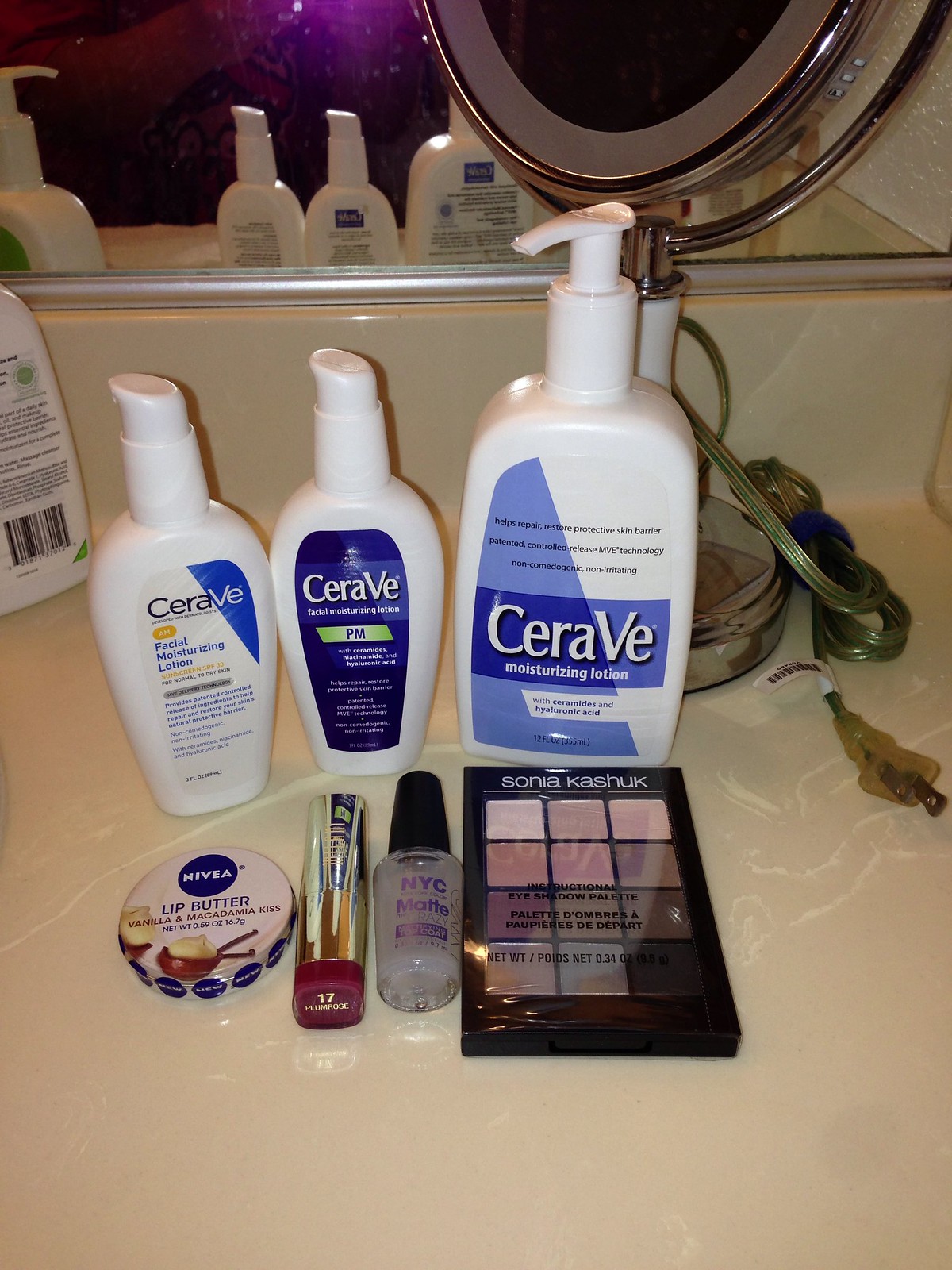In this detailed image, we see a bathroom sink accompanied by various skincare and beauty products meticulously arranged on the countertop. Dominating the scene are three prominent containers of CeraVe products: on the left, CeraVe Facial Moisturizing Lotion; in the center, CeraVe PM; and to the right, a larger tub labeled CeraVe Moisturizing Lotion. Behind these products, a lighted vanity mirror is positioned in front of a larger, basic square mirror, giving the scene a symmetrical backdrop.

To the right of the CeraVe products, we find a neatly placed array of cosmetics. There is a tube of Nivea Lip Butter, identified by its prominent branding. Adjacent to the lip butter is a lipstick, followed by a bottle of clear nail polish labeled NYC Matte. Further right, there is a container housing multiple colors of mascara, adding a vibrant splash to the otherwise minimalist setup. 

In the upper left-hand corner of the image, just partially visible, is another tub of lotion, contributing to the overall theme of skincare and personal care. This detailed composition not only highlights the focal skincare products but also intricately showcases the variety of beauty essentials typically found in a personal grooming space.